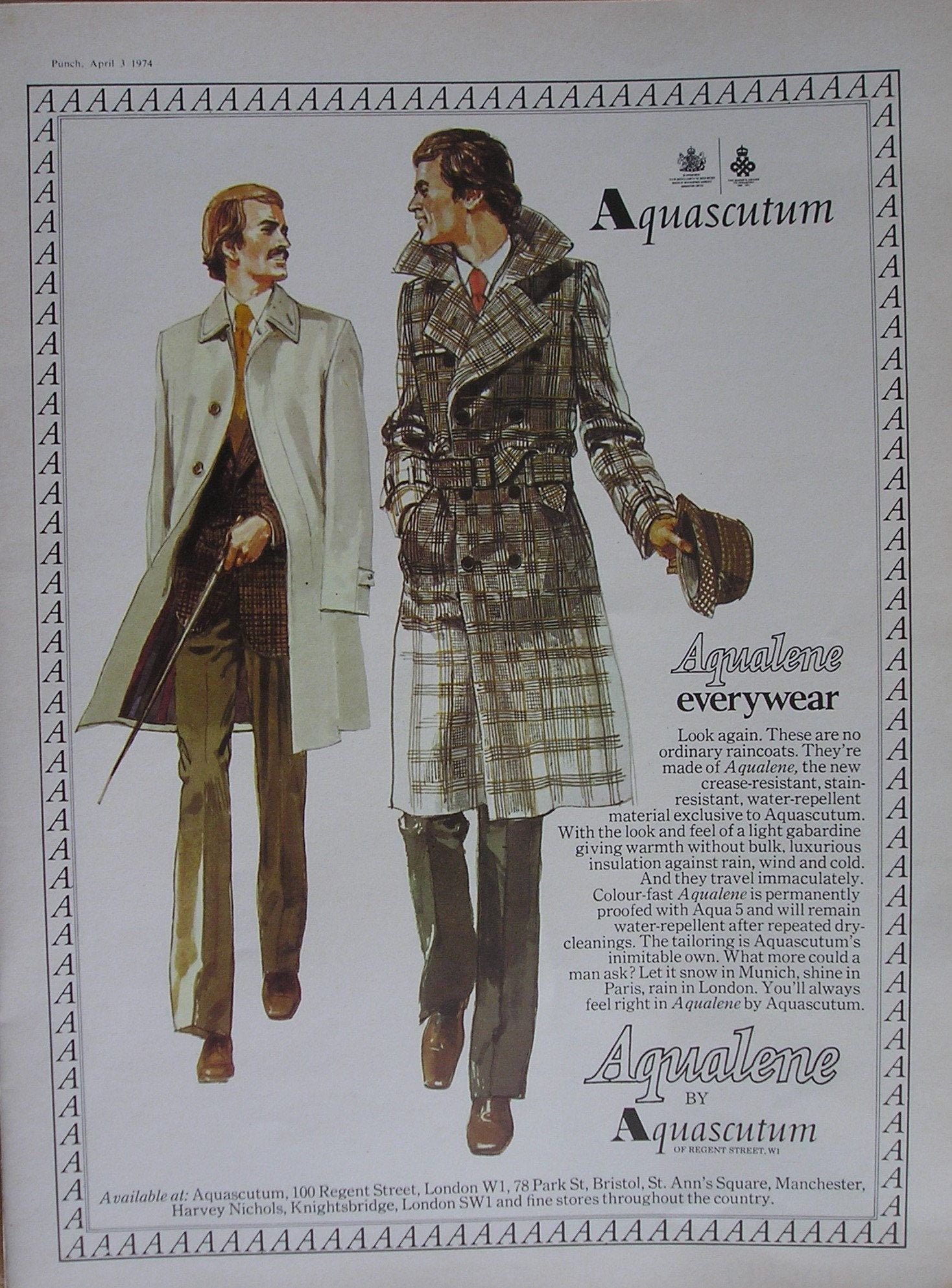This vintage advertisement for Aquascutum showcases an impeccably illustrated scene framed by a border of repeated "A" letters, with "Aquascutum" prominently displayed in the top right corner. At the center, two well-dressed gentlemen are depicted, both wearing sophisticated long coats suitable for colder weather. The man on the left, sporting light brown hair and a mustache, is clad in a solid whitish coat with an orange tie, a brown shirt, matching trousers, and brown boots, and he's holding a pointy stick. The man on the right, with darker hair, wears a checkered coat with a mix of browns and grays, a red tie, dark gray pants, and brown loafers. He also holds a bowler hat. Both men, epitomizing elegance, are engrossed in conversation as they stroll.

The advertisement extols the virtues of Aqualine, a luxurious new fabric exclusive to Aquascutum, known for its crease-resistant, stain-resistant, and water-repellent properties. This extraordinary material maintains its water-repellency even after multiple dry cleanings. Its light gabardine feel provides warmth without bulk, offering ideal insulation against rain, wind, and cold. The impeccable tailoring, synonymous with Aquascutum, ensures the wearer is prepared for any weather—be it snow in Munich, sunshine in Paris, or rain in London. The caption reiterates, "Aqualine by Aquascutum," emphasizing the brand's exclusive innovation in men's outerwear.